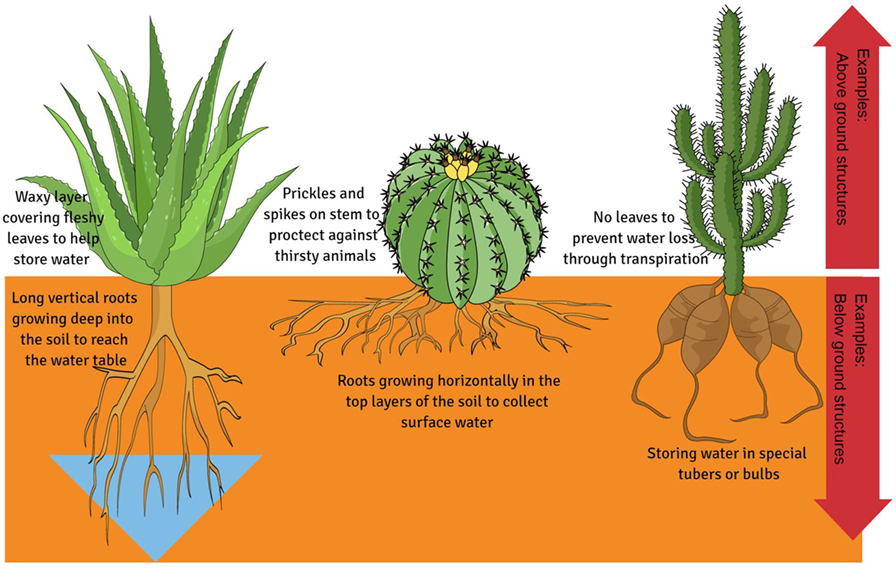This detailed illustration showcases three types of cacti and their unique adaptations for water conservation and protection. The artwork includes an underground cross-section of the soil, depicted as a large brown square, revealing intricate root systems. Beneath the soil, a small blue patch symbolizes the presence of an underground water source.

The first cactus is highlighted with annotations explaining its features: a waxy layer covering its leaves to minimize water loss and long, vertical roots that penetrate deep into the soil, reaching the water table.

The second cactus is characterized by prickles and spikes along its stem, serving as a defense mechanism against herbivores. Its root system spreads horizontally near the surface, optimized for capturing scarce surface water.

The third cactus adaptation described includes the absence of leaves to reduce water loss through transpiration and the ability to store water in specialized tubers or bulbs. Two prominent red arrows accentuate key points of the roots and water storage adaptations.

Overall, the caption emphasizes how each cactus has evolved distinct strategies for surviving in arid environments.